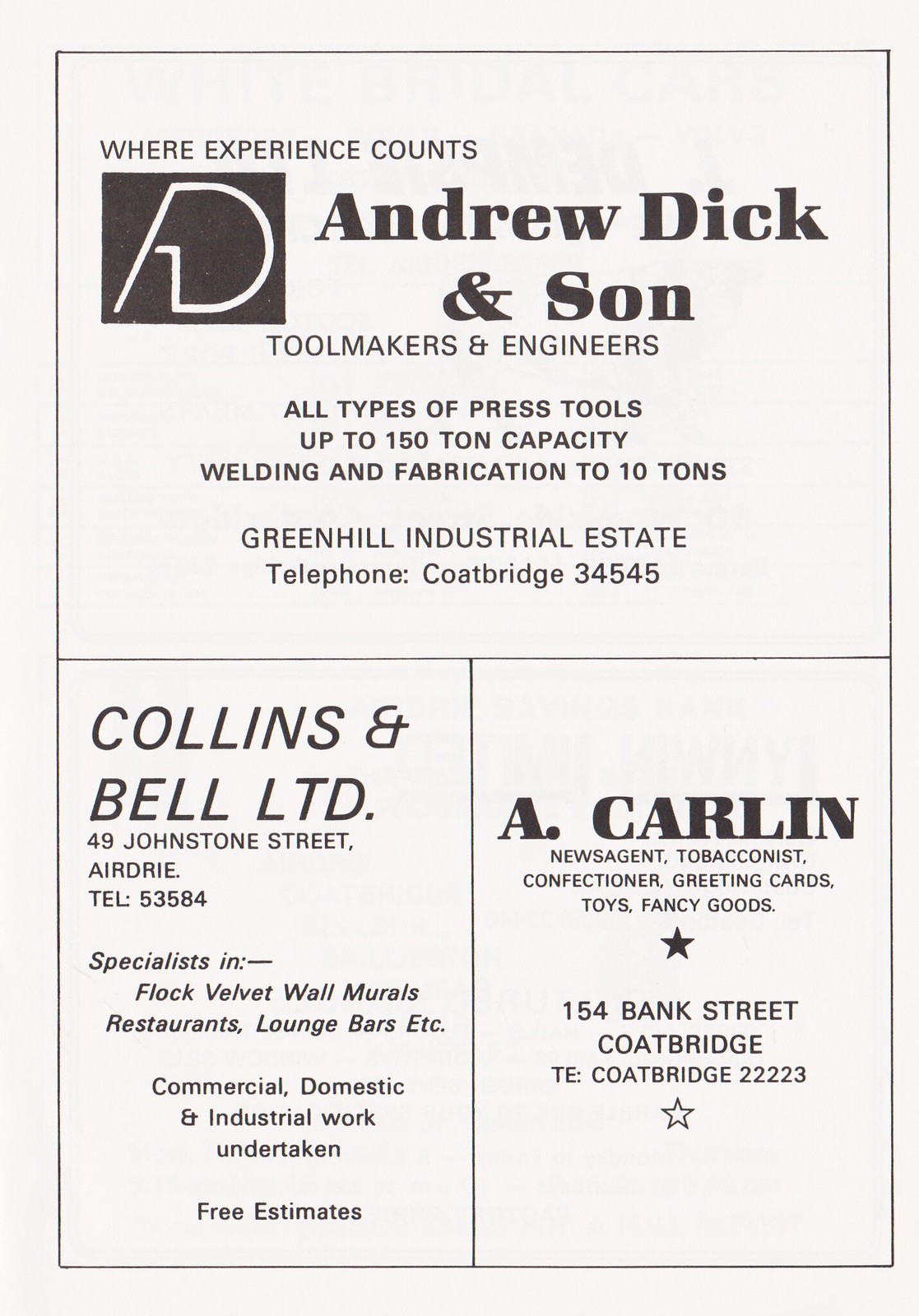The flyer features advertisements for three different businesses against a light gray background, bordered by thin black lines that section the flyer into three parts. The top section highlights the business: "Where Experience Counts - Andrew, Dick, and Son." It includes a logo that combines the letters "A" and "D" and offers services such as toolmaking and engineering, capable of handling press tools up to 150-ton capacity, and welding and fabrication up to 10 tons. The business is located in the Green Hill Industrial Estate, and can be contacted at Cope Bridge 34545.

The lower half of the flyer is divided into two square ads. To the left, "Collins and Bell LTD" at 49 Johnstone Street, Airdrie, offers specialist services in flock velvet wall murals for settings such as restaurants and lounge bars. They undertake commercial, domestic, and industrial projects and provide free estimates. Their contact number is 53584.

On the right, "A. Carlin" advertises itself as a news agent, tobacconist, and seller of confectionery, greeting cards, toys, and fancy goods. Located at 154 Bank Street, Cope Bridge, they can be reached at Cope Bridge 22223. A star mark appears at the bottom of this section, with distinctive black outline and white filling.